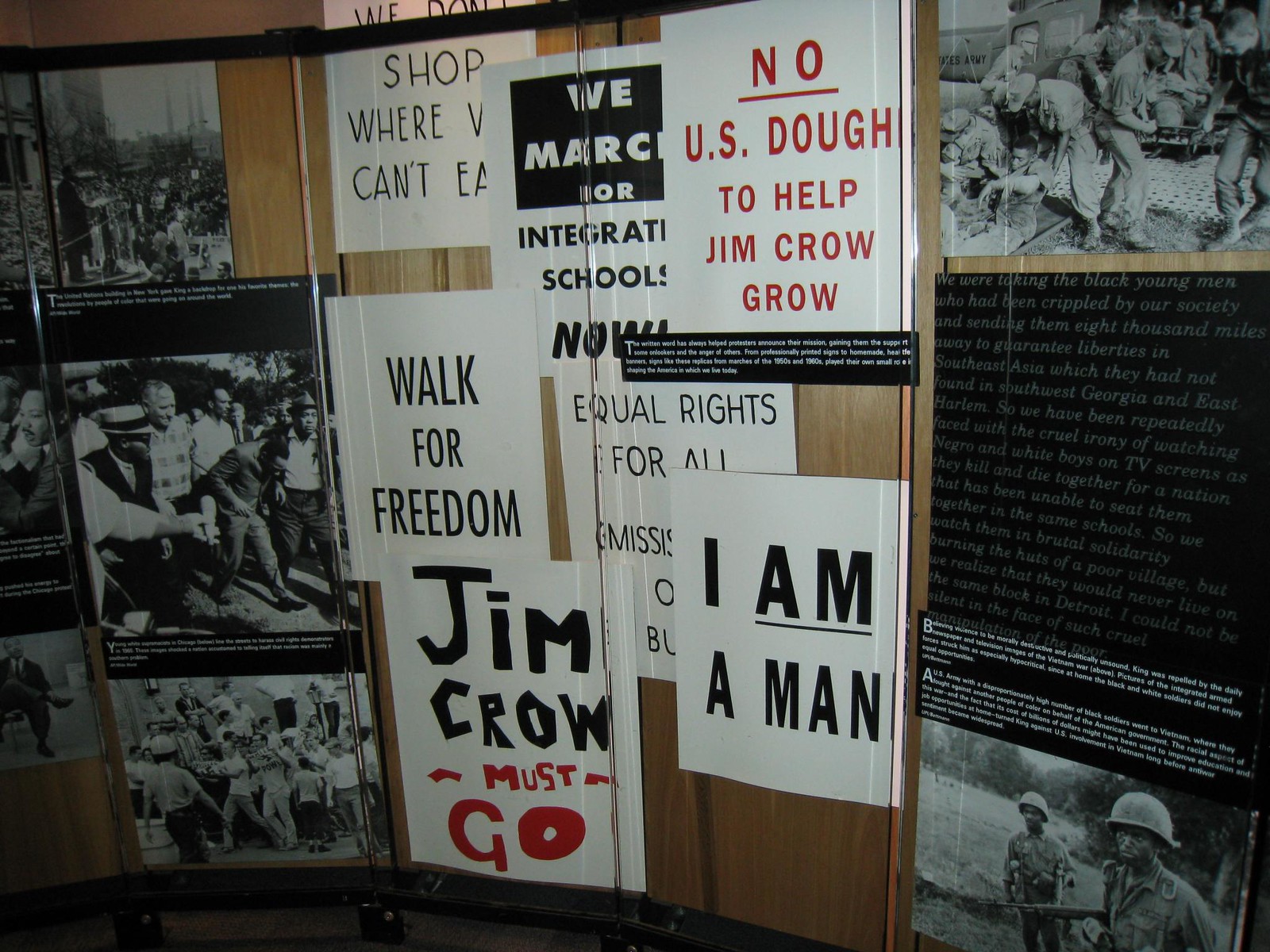The image depicts a detailed museum exhibit enclosed behind glass, showcasing various artifacts from the Civil Rights Movement and the Vietnam War era. Prominently featured are protest signs emblazoned with slogans such as "Jim Crow Must Go," "I Am a Man," "No U.S. Dough to Help Jim Crow Grow," "Walk for Freedom," "We Don't Shop Where We Can't Eat," "Equal Rights for All," and "We March for Integration Schools Now." These signs, mostly in black and white with some hand-done, represent the intense activism against racial segregation.

Adjacent to the signs, there are black-and-white photographs documenting significant moments in the Civil Rights Movement, including images of African American protestors, brawls and riots, riot police, and a possible speech by Martin Luther King Jr. Additional photographs depict the Vietnam War, showing African American soldiers in military uniforms, some emerging injured or deceased from Army helicopters.

The exhibit's backdrop includes detailed scenes of Vietnam, particularly Hanoi, paired with explanatory text. This juxtaposition of Civil Rights memorabilia and Vietnam War imagery captures the turbulent and intersecting historical narratives of the 1960s, emphasizing the era's fight for racial equality and the global conflicts impacting American society.